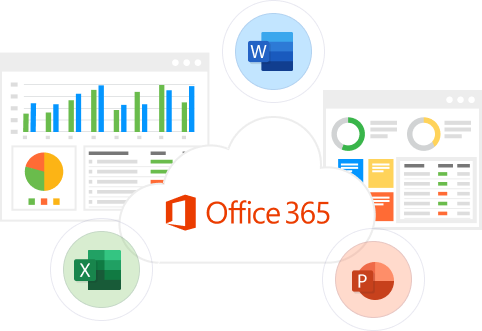This image showcases the suite of Microsoft Office icons prominently in the foreground. The recognizable blue "W" represents Microsoft Word, the green "X" denotes Microsoft Excel, and the orange "P" signifies Microsoft PowerPoint. In the background, a collection of vibrant visuals provides additional context. Colorful pie charts, displaying slices in yellow, yellow-green, and red, add depth and variety. Additionally, assorted icons and circular graphics in different colors, including a notable yellow circle, populate the scene, enriching the overall composition with a dynamic and visually engaging layout.